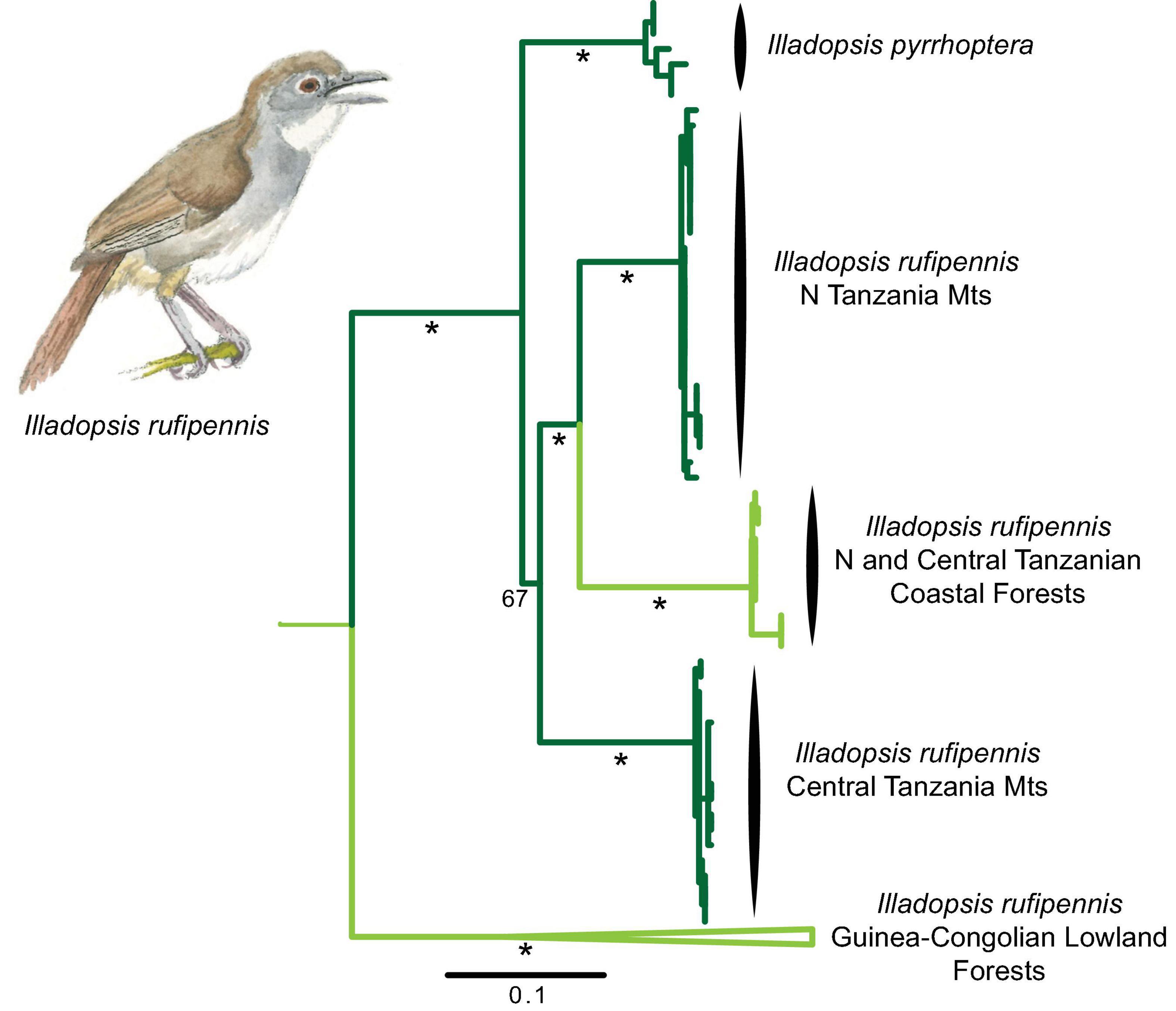The illustration features a detailed, Audubon-style depiction of a bird labeled as "Illadopsis rufipennis." The bird is small, primarily brown with grayish-brown wings and a brown back and tail. Its breast and chin are white, and it has a gray beak slightly open, posed gripping a branch. To the right of the bird is an intricate lateral family tree graph, detailing the bird's scientific classification and geographical distribution. The graph expands horizontally from left to right, becoming increasingly complex. It lists various subspecies and locations: "Illadopsis pyrrhoptera," "Illadopsis rufipennis in Tanzania MTS," "Illadopsis rufipennis North and Central Tanzanian Coastal Forests," "Illadopsis rufipennis Central Tanzania Mountains," and "Illadopsis rufipennis Guinea-Congolian Lowland Forests," suggesting diverse habitats and possibly migration patterns or evolutionary lineage. The image is rich in textual information, featuring names and scientific designations that elaborate on the bird's range and classification.